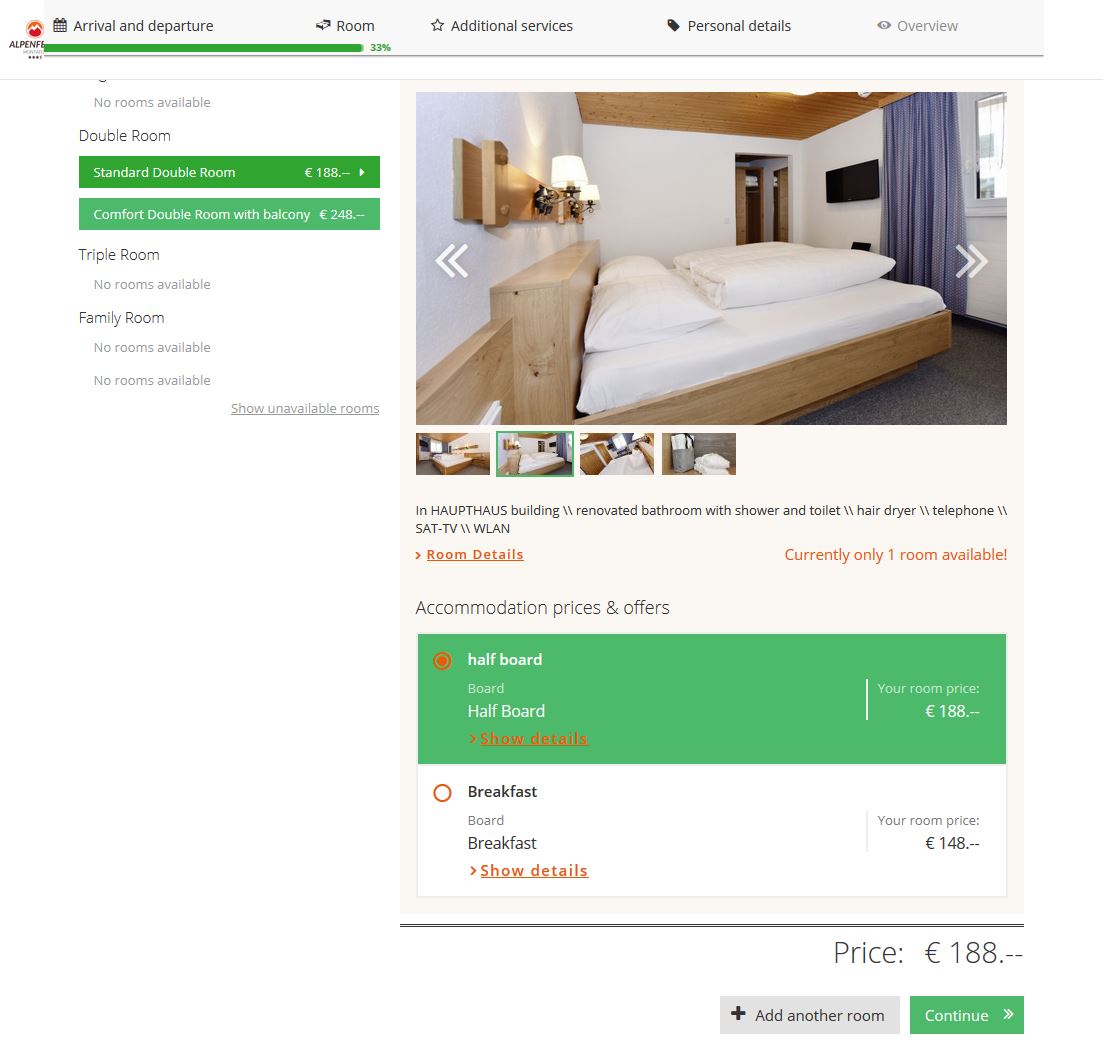Screenshot of the Alpenfee Booking Website

This image showcases a screenshot of the Alpenfee website, designed for booking hotels and flights. At the very top, there's a small, prominent red icon representing the website's logo, accompanied by the site name "Alpenfee." Below that, navigation tabs labeled "Arrival and Departure," "Room," "Additional Services," "Personal Details," and "Overview" guide the user through the booking process. 

A long green progress bar indicates that the user has completed 33% of the booking procedure. On the left-hand side, the room availability is outlined: 

- "No rooms available"
- "Double Room"

Below this, two green rectangular boxes present room options:

- "Standard Double Room"
- "Comfort Double Room with Balcony"

Further down in black text, other room categories are listed, but they are marked as unavailable:

- "Triple Room" (no rooms available)
- "Family Room" (no rooms available)

An option labeled "Show Unavailable Rooms" follows these listings.

On the right side of the image, there's a photograph of a hotel room featuring a bed with white pillows, a brown headboard, white bedside lights, and blue curtains framing a window that offers a glimpse of the outside. Accompanying the image is detailed information about the room.

Additionally, there are two green and white rectangular bars indicating meal options:

- "Half Board"
- "Breakfast"

A price button prominently displays the rate of "88," and there are buttons labeled "Add Another Room" and "Continue" to proceed with the booking process.